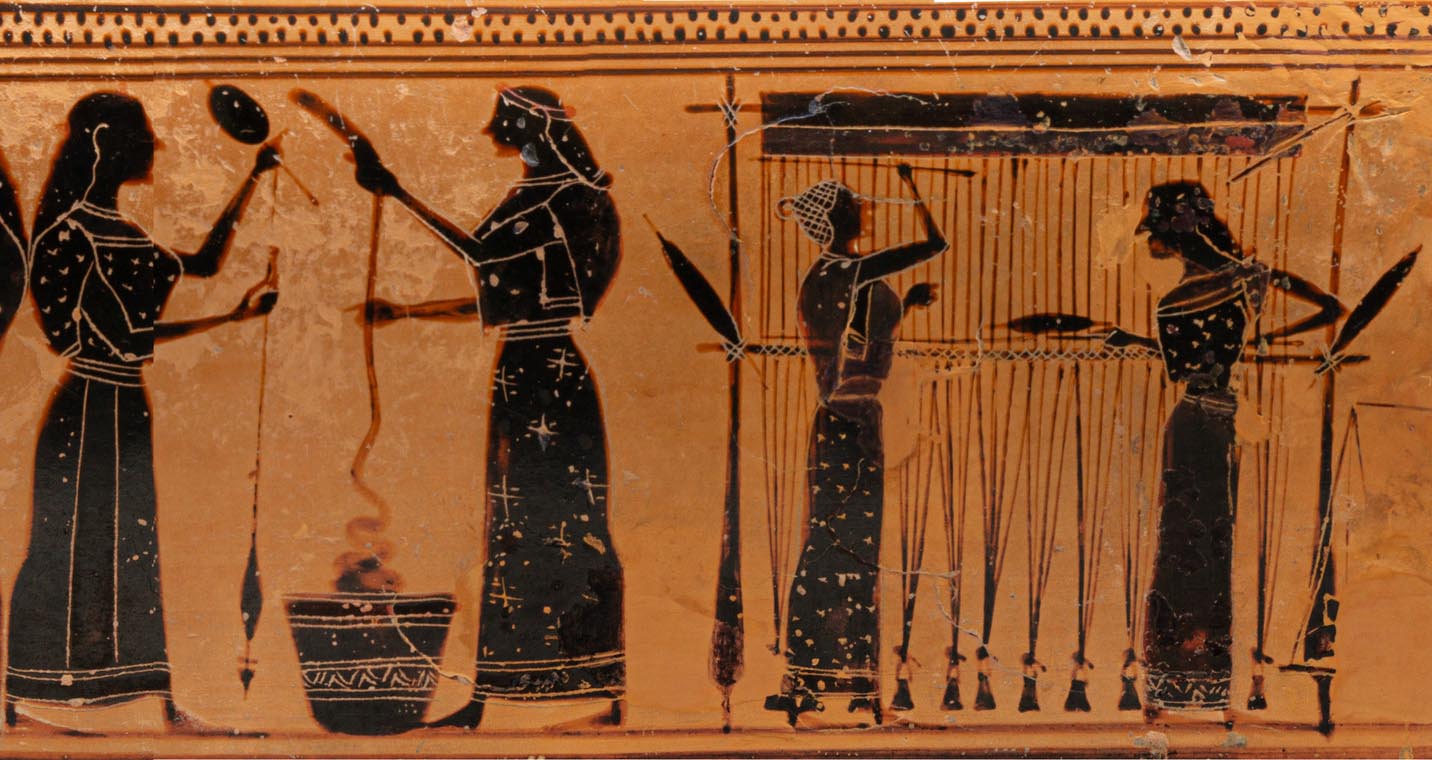The image is an illustration of ancient art, likely inspired by both Egyptian and Greek traditions. The background is predominantly orange with black figures, reminiscent of the decorative styles seen on ancient pottery or wall art. Starting from the left, there are two images of individuals—one holding a long, straight object and the other with a long, crooked item. Moving to the right, two women are seen engaged in textile activities, possibly tending looms for fabric making. The artwork depicts ancient women intricately involved in textile work, which may include weaving, dyeing clothes, or making threads. The scene portrays a detailed snapshot of the ancient world, blending visual elements from both Egyptian and Greek artistic cultures.